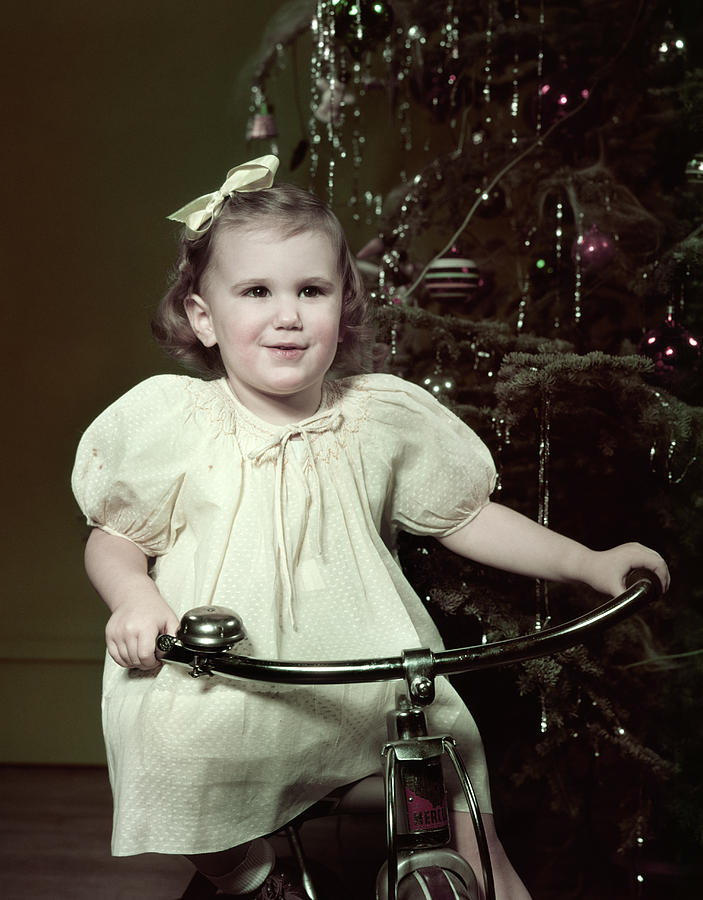A vintage photograph showcases a cheerful Caucasian little girl, positioned towards the left of the image, sitting on a classic red bicycle in front of a richly decorated Christmas tree, evocative of the 1950s. She is adorned in a pale chiffon dress with smocking around the neck and a delicate bow, complemented by a bow in her short brown hair. Her bright smile and hands firmly grip the curved metal handlebars, which feature a small bell. The background reveals a large evergreen tree, adorned with tiny lights, tinsel, silver garland, and an array of ornaments in red and maroon hues, standing beside a white wall and wooden floor, grounding the festive setting.